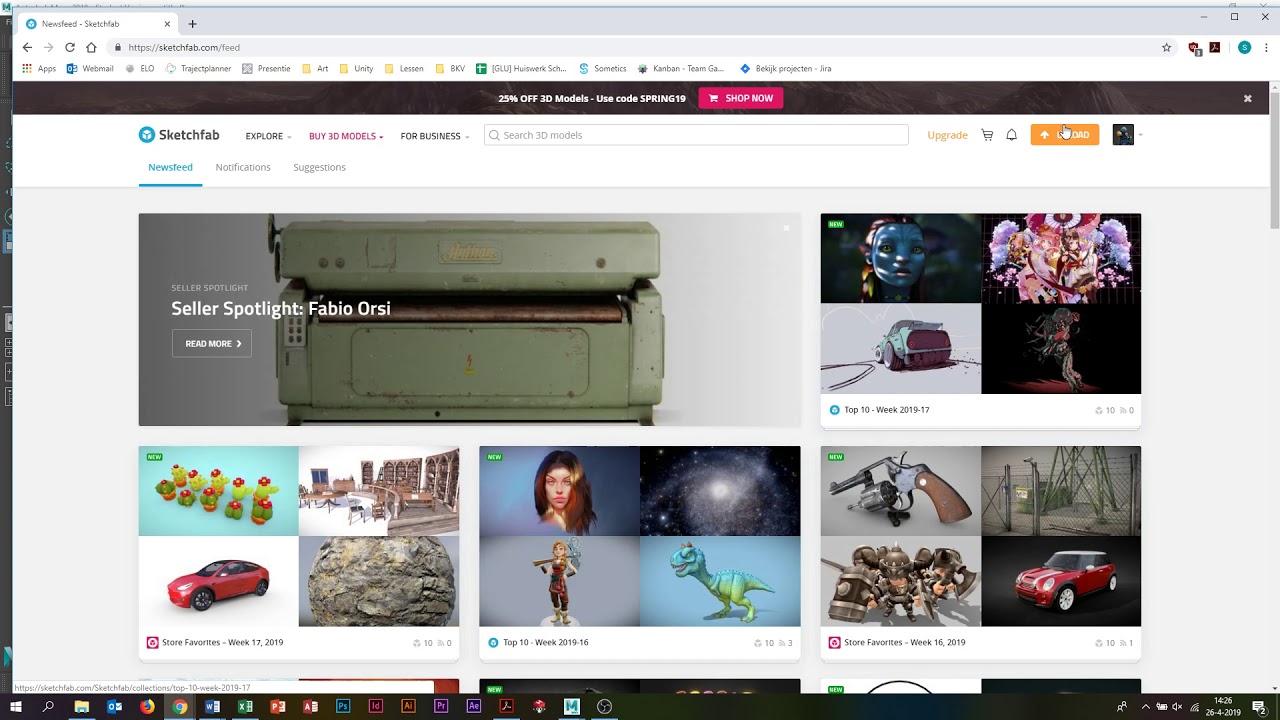This screenshot captures a web page from Sketchfab, specifically the 'Newsfeed' section, as indicated by the underlined "Newsfeed" in the top navigation bar, along with adjacent tabs for "Notifications" and "Suggestions." The URL bar clearly displays "sketchfab.com/feed."

The main content area features a series of boxed images that are part of the feed. One prominent section is titled "Seller Spotlight: Fabio Orsi," accompanied by a "Read More" link for additional information. Further down, there are highlighted categories such as "Store Favorites" with entries like "Top 10 Week 2019-16" and "Top 10 Week 2019-17," along with a specific mention of "Store Favorites Week 16, 2019."

Near the top right, there is an orange box containing options for "Upload," "Download," and "Upgrade," designed for user interactions. This section is distinguished by its bright color, making it easy to spot for quick access.